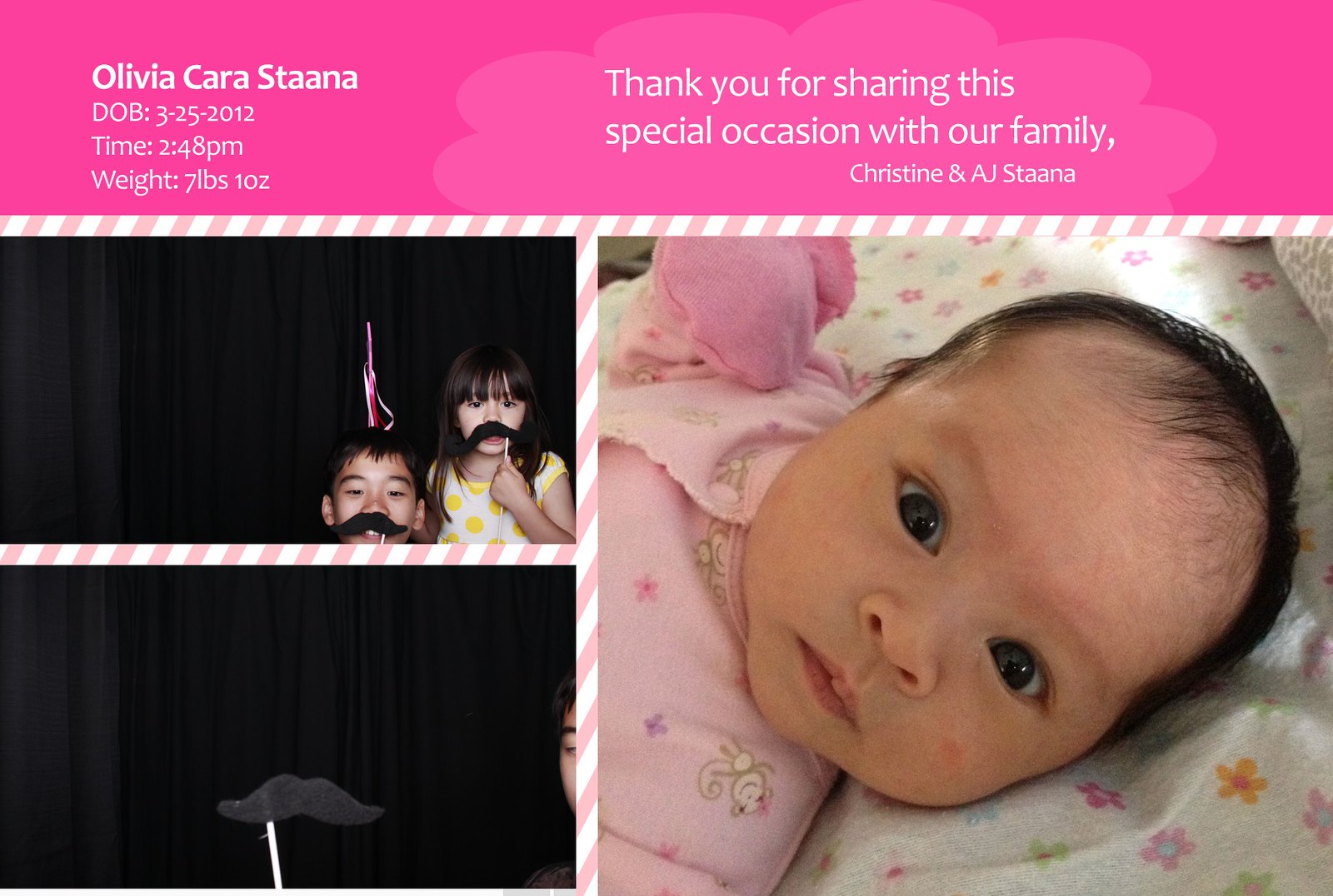The image is a thoughtfully composed combination of color photography and graphic design in a horizontal, rectangular format, creating an elegant card. At the top, a horizontal pink strip spans about a quarter of the image's height. On the left within this strip, it reads "Olivia Cara Stana, DOB 3/25/2012, time 2:48 PM, weight 7 pounds, 1 ounce" in white text. On the right, also in white text within the pink strip, it says, "Thank you for sharing this special occasion with our family, Christine and AJ Stana."

Below this pink band, the lower right section features the largest photo—a square image of Olivia as a baby. She has dark hair, is wearing pink pajamas, and lies in a crib with white floral sheets, gazing up at the camera. To the left, there are two smaller, horizontal photographs. The top left photo shows Olivia at an older age, playing with her brother while both don fake mustaches, smiling towards the camera. Beneath it lies another horizontal photo, which is a close-up of just the fake mustache on a stick against a dark background.

The essence of the image is enhanced by a range of colors, including pink, black, yellow, white, purple, gray, and cream, contributing to its warm and inviting aesthetic. The photos appear to have been taken indoors, with the largest one on the right seemingly captured during the day. This well-designed composition blends representational photography with graphic elements to create a cherished memento.